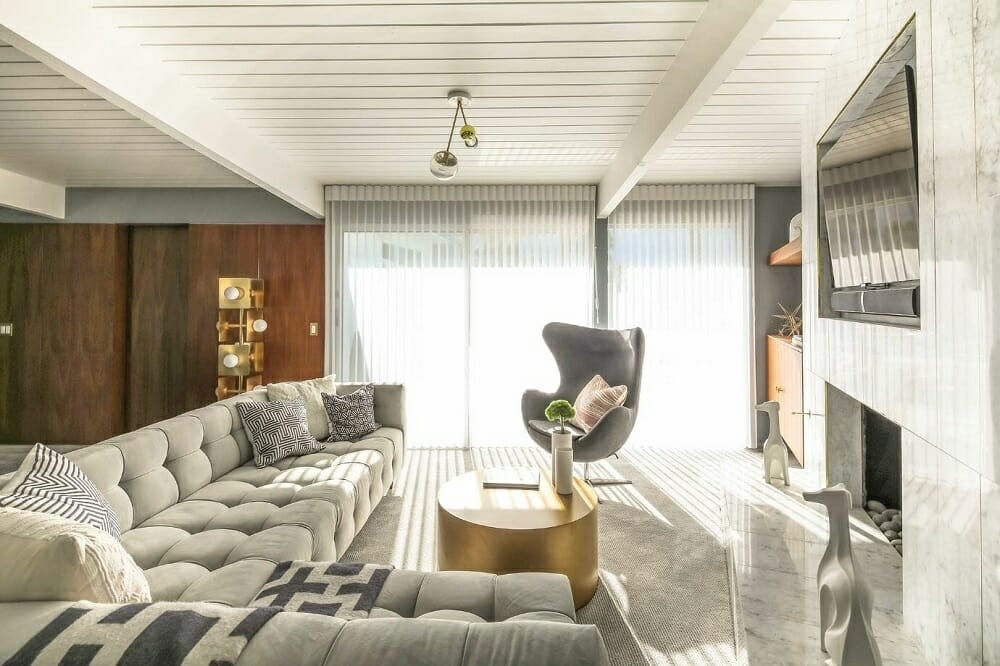This photograph showcases a stylish, modern living room with a touch of retro 1970s flair. Dominating the right side of the room is a striking large fireplace made of marble-like stone, its base adorned with two detailed stone carvings of large dogs and lava rocks. Above the fireplace, a built-in section houses a flat-screen TV and a soundbar, with the TV slightly tilted. The floor is covered in a tightly woven white carpet, adding a clean and soft texture to the space. 

On the left side of the room, a spacious gray sectional couch, arranged in an L-shape, is beautifully accented with patterned white and dark gray pillows, as well as a gray and white blanket draped casually over the back. A small, round gold coffee table centered in the room features a book and two cylindrical vases that hold small green flowers, adding a touch of freshness to the setting. 

A large, rounded gray chair reminiscent of the 1970s TWA airport lounge style sits prominently, adding to the retro vibe that permeates the space. The wood-paneled wall in the background, composed of dark wood, contrasts with the ceiling’s white wood paneling and white beams, creating a harmonious blend of textures and colors. 

The room is well-lit by a large sliding glass door fitted with floor-to-ceiling white blinds. Adding a splash of eclectic charm, a gold floor lamp designed to look like a series of boxes with round bulbs stands gracefully. This carefully decorated living area brings together modern sophistication with nostalgic elements, creating a unique and inviting ambiance.